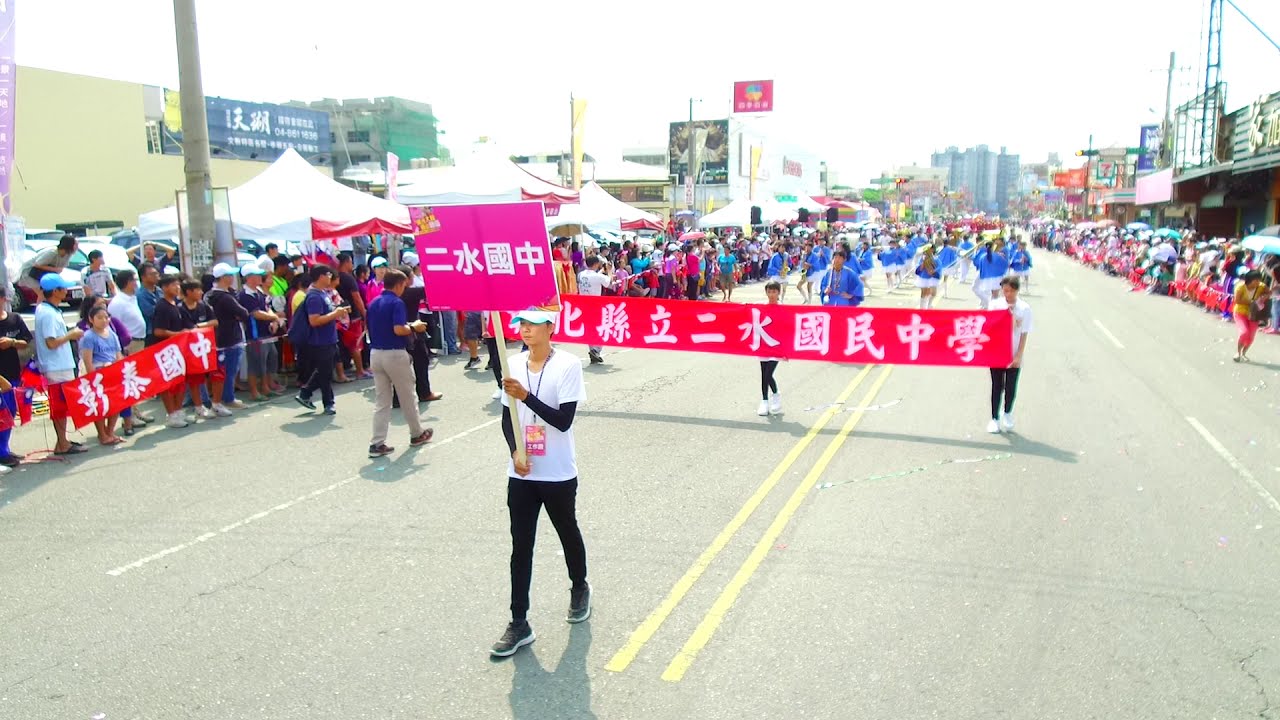This detailed landscape-oriented color photograph captures a vibrant street parade marching through a city avenue. Leading the parade is a gentleman dressed in a white t-shirt layered over a black long-sleeve shirt, paired with black pants and black and white shoes. He wears a green hat and a long necklace adorned with a badge. Holding a red sign with white Asian symbols on a light-colored wooden stick, he commands attention as he walks down the center of the closed, paved roadway. Just behind him, three individuals, dressed similarly in white shirts, black pants, and white shoes, hold up a horizontal red banner also inscribed with white Asian symbols. Following them, a group of participants dressed in matching blue tops and white bottoms, possibly cheerleaders, wave rods in their hands. The parade proceeds along streets lined with a mix of storefronts and taller buildings in the hazy, sunlit background. Bystanders crowd both sides of the street, cheering on the procession, contributing to the lively atmosphere of this urban celebration. The photograph is taken from a low vantage point, possibly by a drone, adding a unique dynamic to the scene captured in photographic representationalism.